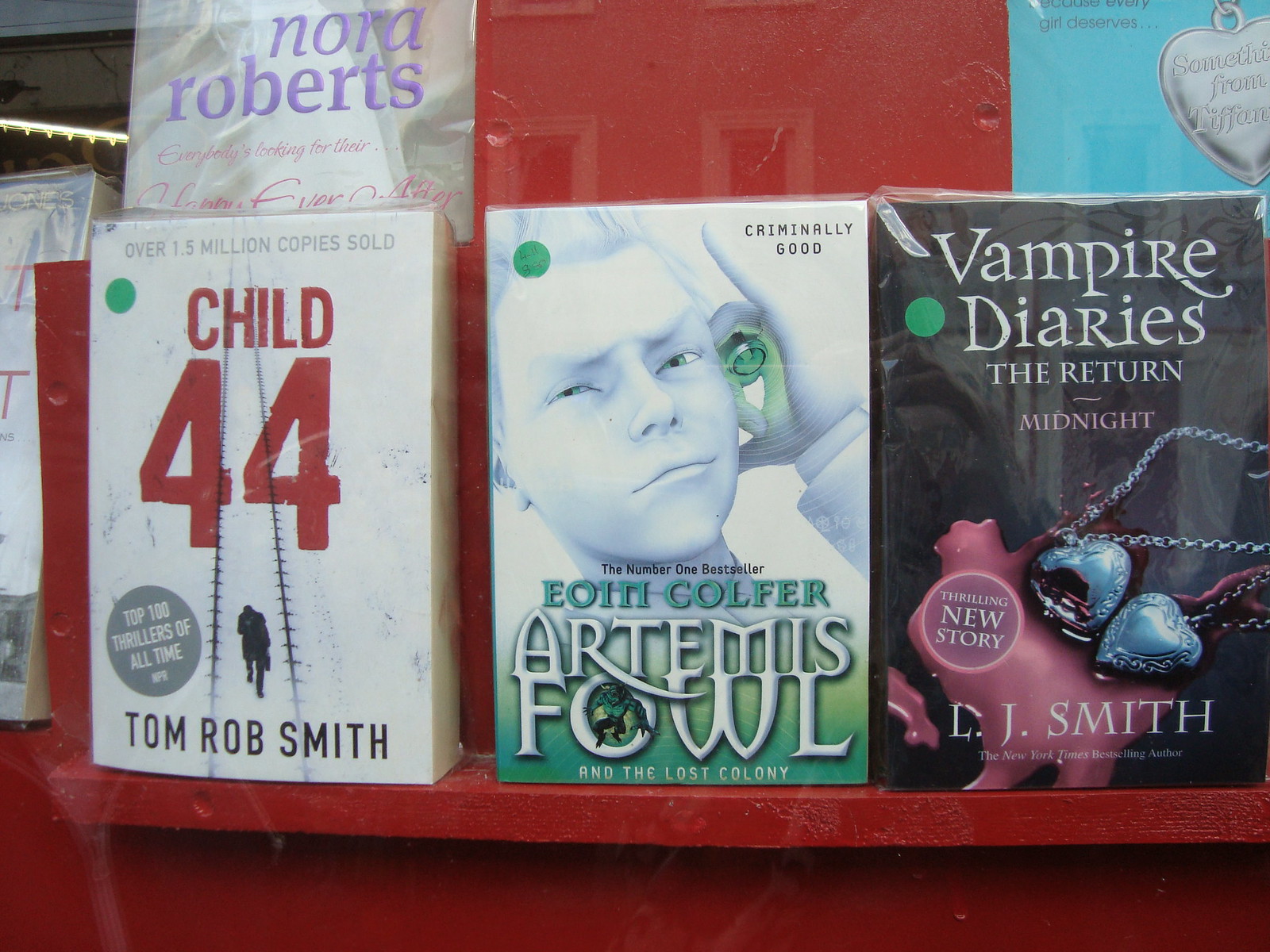The photograph captures a vibrant window display featuring a three-tiered red shelf filled with a selection of upright books, set within a glass case likely found in a store. On the top left corner, a book by Nora Roberts prominently features her name in purple with a pink cursive script underneath. On the lower left shelf, there's a white-covered book advertising "Over 1.5 million copies sold." In red, it showcases "Child 44" by Tom Rob Smith, adorned with an image of a staircase and a man ascending it. To its right, a book with a white jacket displays a sketch of a green-eyed man's face, with "Eoin Colfer" in green ink and "Artemis Fowl and the Lost Colony" in white font. Adjacent on the right, a black-covered book titled "Vampire Diaries, The Return: Midnight" in white font features a locket and a pool of blood, authored by L.J. Smith. In the upper right corner, a turquoise book partially cut off by the camera shows a silver locket, with unclear additional details. Reflective elements on the window add depth to this meticulously arranged literary display.